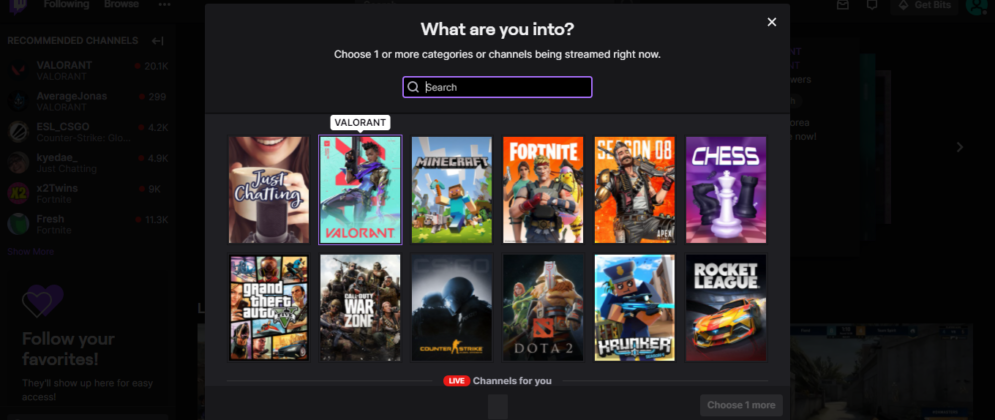The image displays a prominent gray window overlaying a partially obscured background screen. The background screen is heavily grayed out, rendering its contents largely unreadable, except for a few visible names and numbers. Below this, three icons and a message are discernible: a purple heart, a white heart, and text that reads, "Follow your favorites, they'll show up here for easy access."

At the top of the gray overlay, the header reads "What are you into?" accompanied by a close button (X). Below, instructions invite users to "choose one or more categories or channel to be streamed right now." 

Directly beneath these instructions is a black text box with a purple border, featuring a magnifying glass icon and the word "Search." Further down are six movie thumbnails displayed in a two-row grid. From left to right on the top row, the thumbnails are labeled "Just Chatting," "Valorant," "Minecraft," "Fortnite," an unclear title, and "Chess." On the bottom row, the thumbnails are labeled "Grand Theft Auto V" and "Warzone."